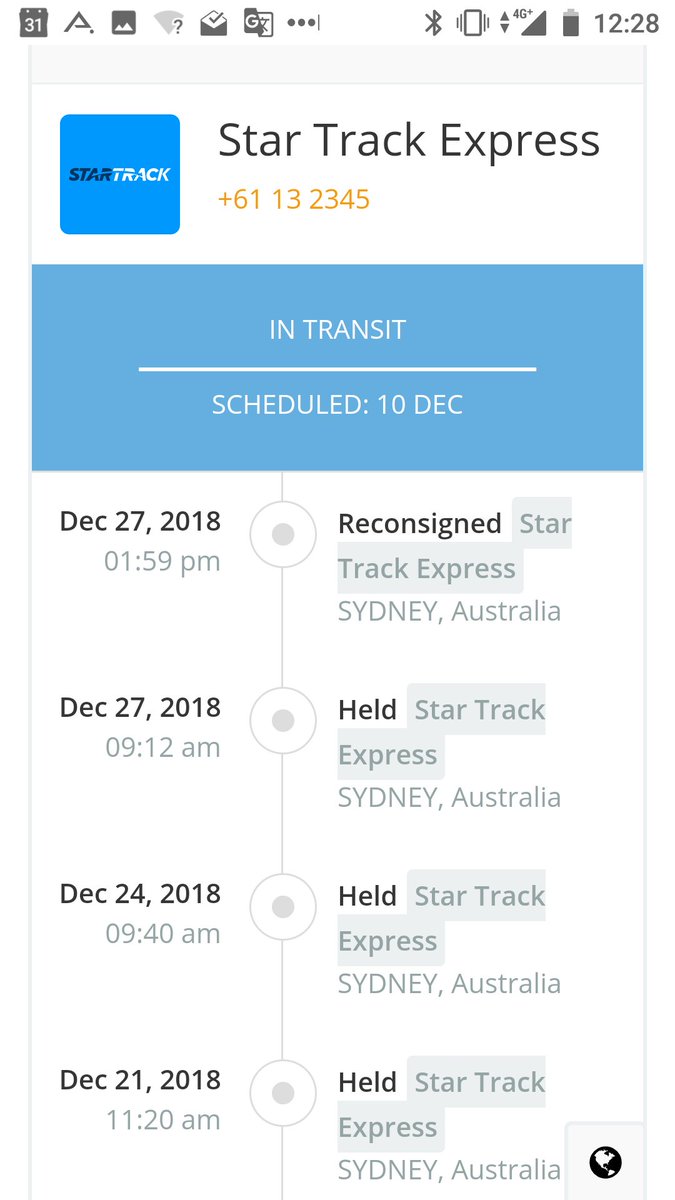The image displays the tracking information for a delivery service called StarTrackExpress, presented within a blue panel at the center of the screen. The status indicates that the shipment is "In Transit" and was initially scheduled for delivery on December 10th. However, the delivery attempt was unsuccessful on that date. Following this, the package was held multiple times: on December 21st, 24th, and again on the 27th. Later on December 27th, at 1:59 p.m., the parcel was marked as "Re-Consigned," indicating its relocation for another delivery attempt.

In the upper section of the screen, several icons common to a Google-based smartphone interface are visible. These include a calendar icon, a Bluetooth symbol, 4G network signal strength, and the battery indicator, which shows a substantial amount of battery life remaining. The device's clock displays the time as 12:28. This detailed tracking update reflects the complexities and delays that have impacted the delivery process, resulting in an extended and unresolved shipment status.